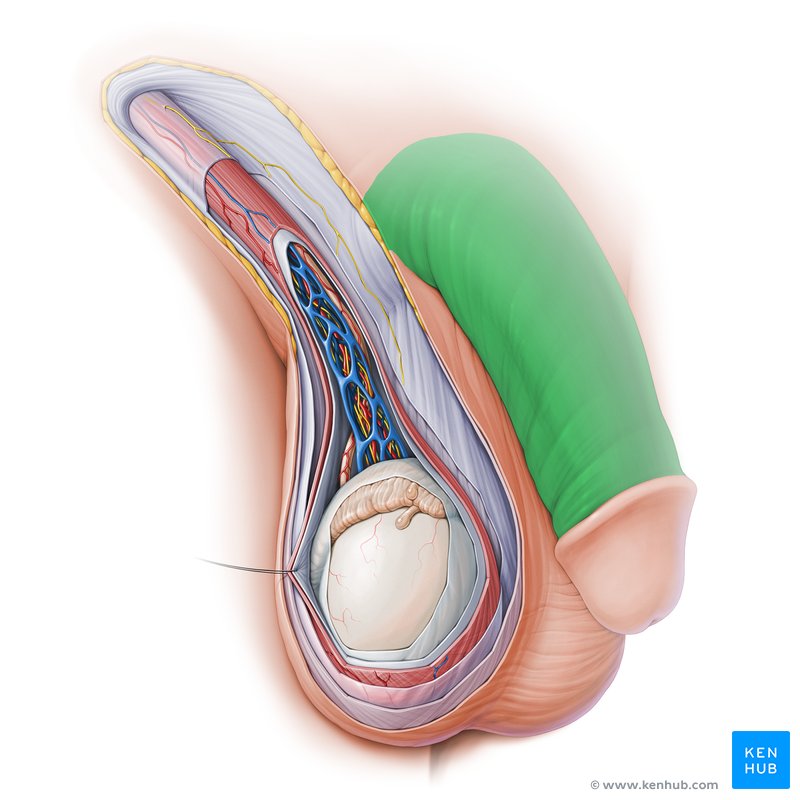The image appears to be a detailed, medical drawing of the male reproductive system, resembling those found in an anatomy textbook. The illustration prominently features the penis and testicles, with the penis rendered in green, except for the flesh-colored tip. On the right side, the drawing reveals an intricate view of the interior of the testicle, showing various veins, capillary blood vessels, nerve endings, and different layers of tissue, depicted in colors such as white, red, purple, and blue. The spongy-looking tissue can be observed, along with the wrinkle-like texture of the outer skin of the testicles. The image extends from the lower abdomen, likely showing part of the bladder, down to the detailed internal structure of the testicles. The anatomical accuracy, intricate details, and the 3D perspective indicate that this is a scientific medical illustration. The bottom of the image bears a copyright notice for Ken Hub with their website and logo.